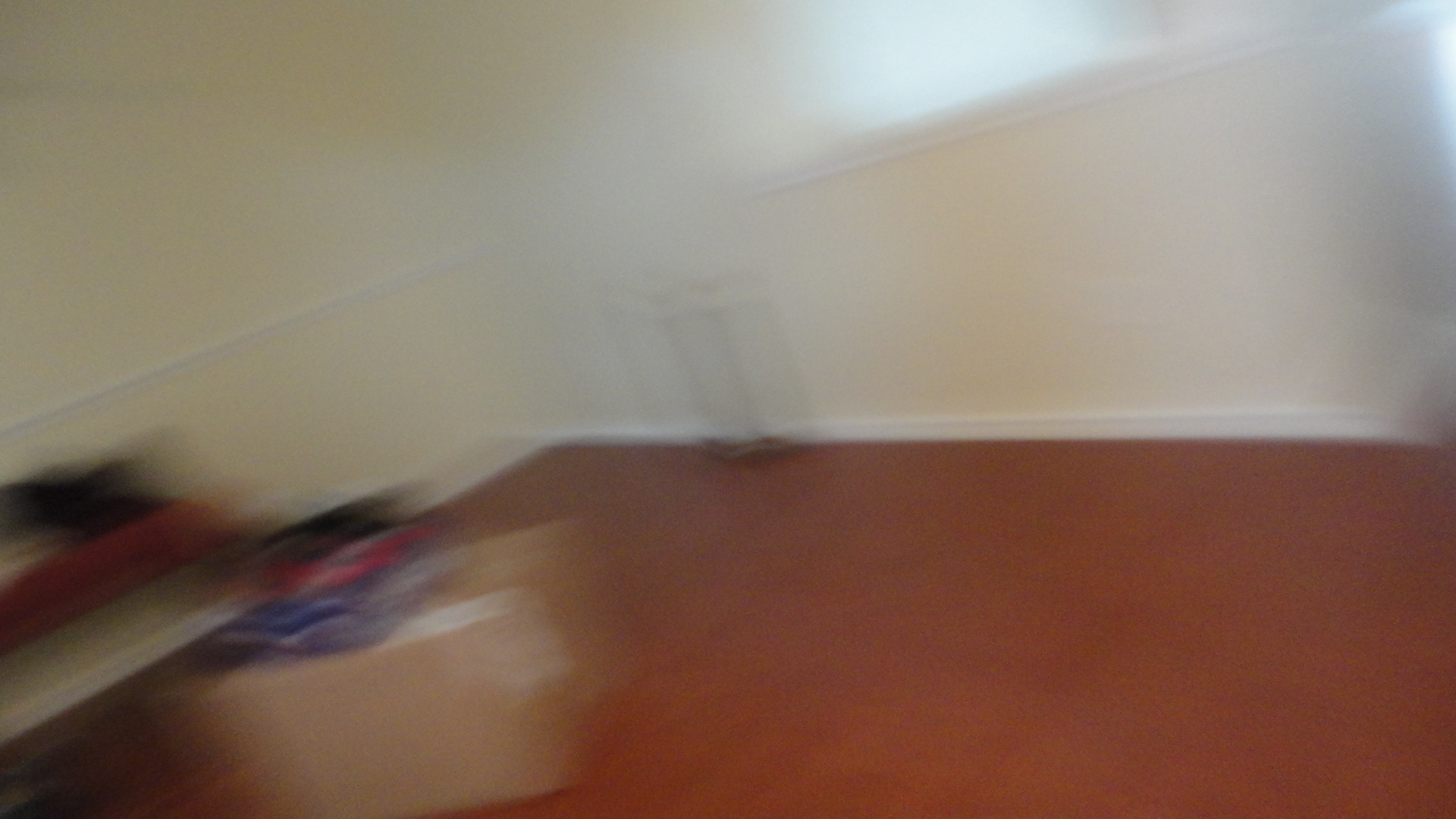The photograph, captured amidst significant motion blur, depicts the corner of a room with light tan or yellowish cream-colored walls. The image is angled in a disorienting manner, leading to a skewed perspective that emphasizes the lower portion of the scene. The floor appears to have a reddish hue, possibly made of wood or covered with a fabric material. In the bottom left corner of the image, there is a box-like object on the ground, with what seems to be a white coffee table slightly to the right of it. Further to the right, there's a piece of furniture, potentially a couch or chair, though it's also difficult to discern due to the blur. The right wall features a partially visible window, which casts a bright glare from the sunlight streaming through it. A skirting board is noticeable where the walls meet the floor, adding a subtle trim to the room's decor.